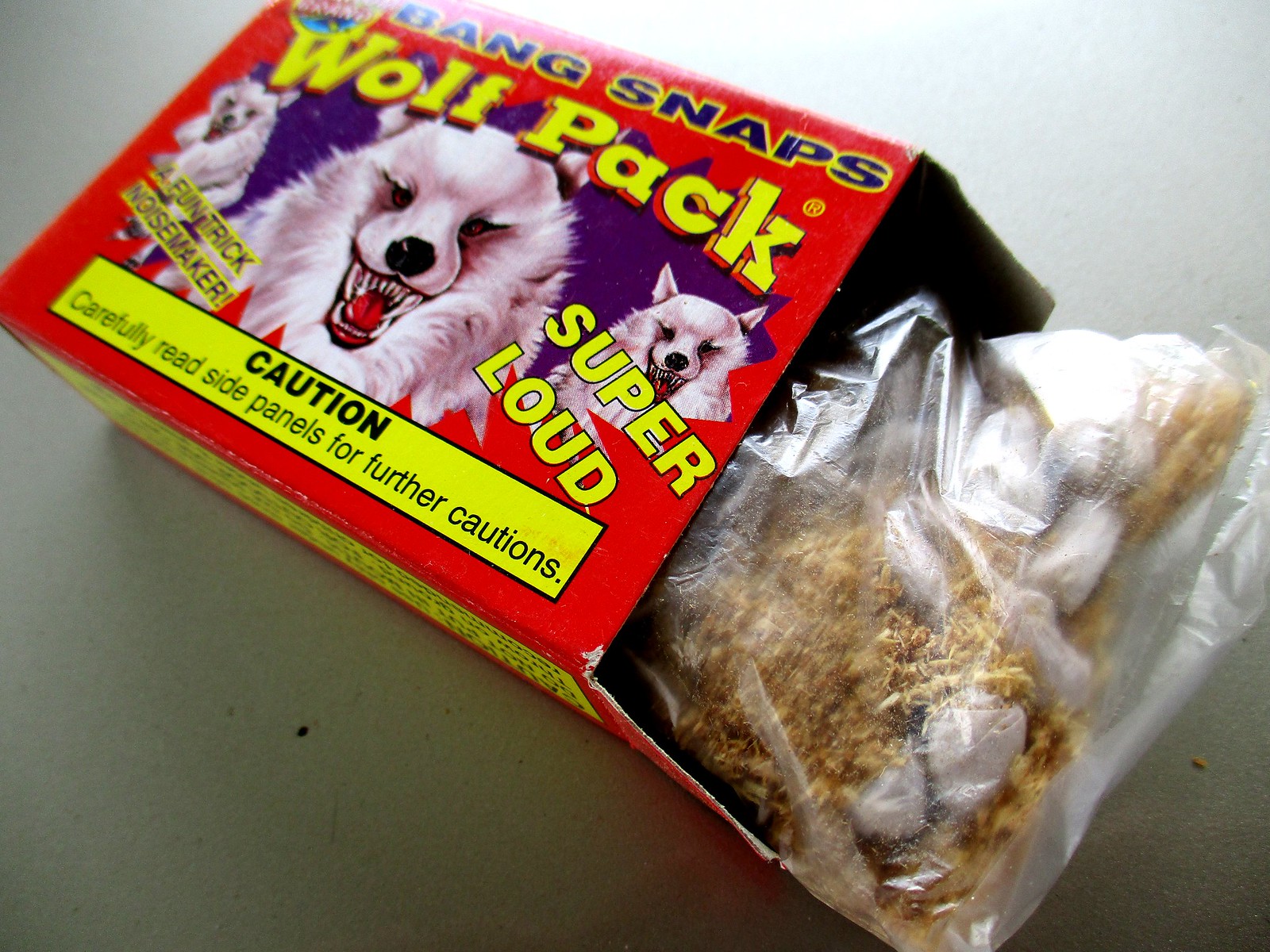This image shows an open red box labeled "Bang Snaps Wolf Pack" with three illustrations of snarling white wolves. The text on the box boasts "Super Loud" and describes the contents as a "Fun Trick Noisemaker." A warning at the bottom advises, "Caution: Carefully read side panels for further caution." Inside the box, white paper-wrapped firecrackers, also known as snaps, are nestled in sawdust packing within a plastic bag. These snaps are typically thrown on the ground where they make a popping noise, commonly associated with celebrations like the 4th of July. The scene is illuminated by natural-looking light, possibly from a nearby window, creating a bright setting on a grayish table.